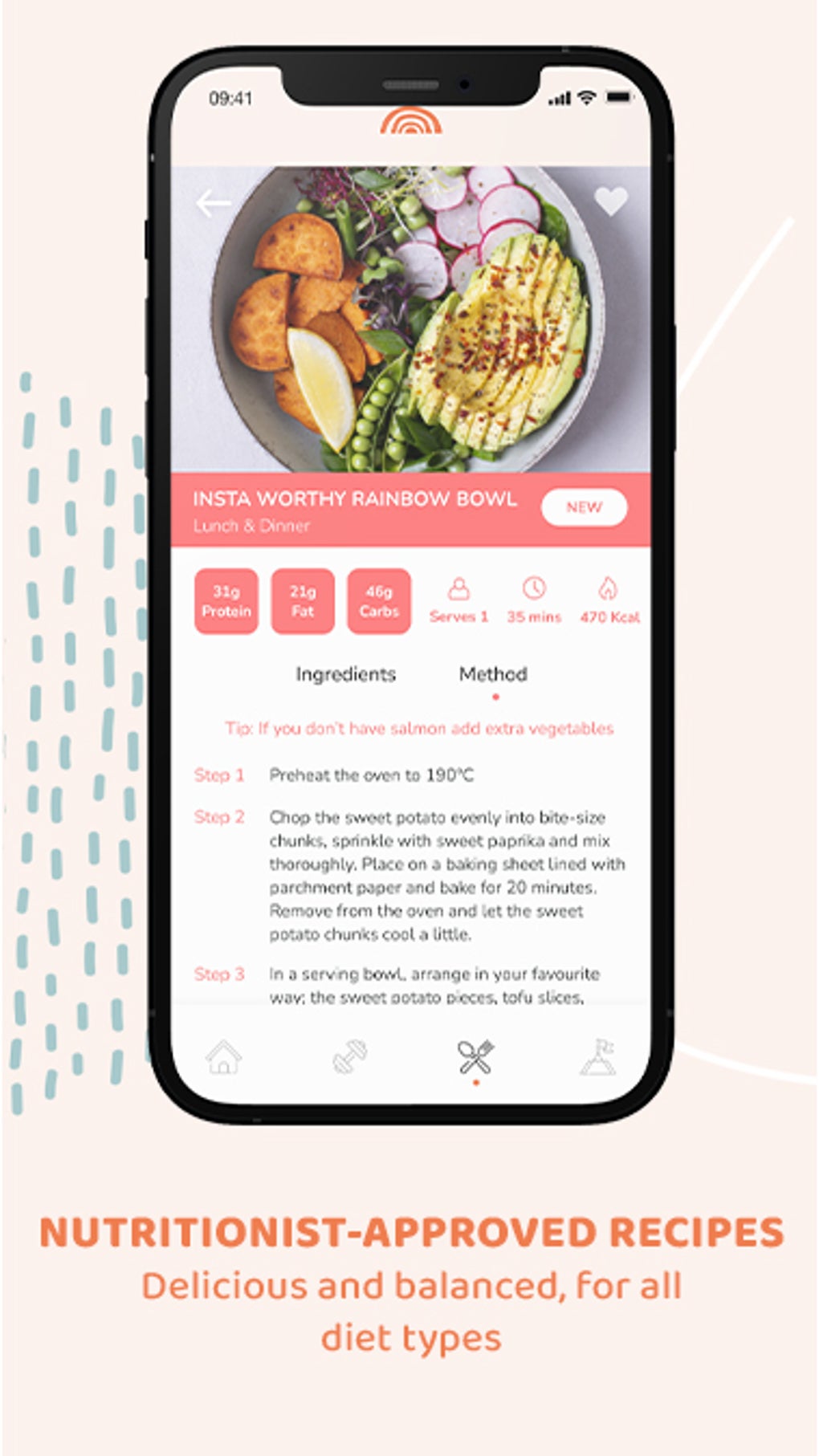The image is a screenshot of a website advertisement featuring a smartphone against a beige background. The smartphone has black bezels and a photoshopped screen. The top left corner of the screen displays the time, 9:41, while the top right corner shows icons for full WiFi, mobile signal, and battery.

The main content of the smartphone screen begins with a photograph of a vibrant bowl of food at the top, featuring sliced avocado, soybeans, a sliced egg, and radishes. Directly below this image, a pink bar with white font reads "Insta-worthy Rainbow Bowl." It also indicates that the dish is suitable for both lunch and dinner, with a "new" button to the right.

Further down, there are three pink boxes with white text detailing the nutritional information: 31g of protein, 21g of fat, and 45g of carbs. The dish serves one, takes 35 minutes to prepare, and contains 470 kcal. Below this in black font, the section labeled "Ingredients and Method" is displayed, with "Method" selected. 

In pink font beneath this, there is a tip suggesting that if you don't have salmon, you can add extra vegetables. The first step of the recipe is then listed: "Preheat the oven to 190°C."